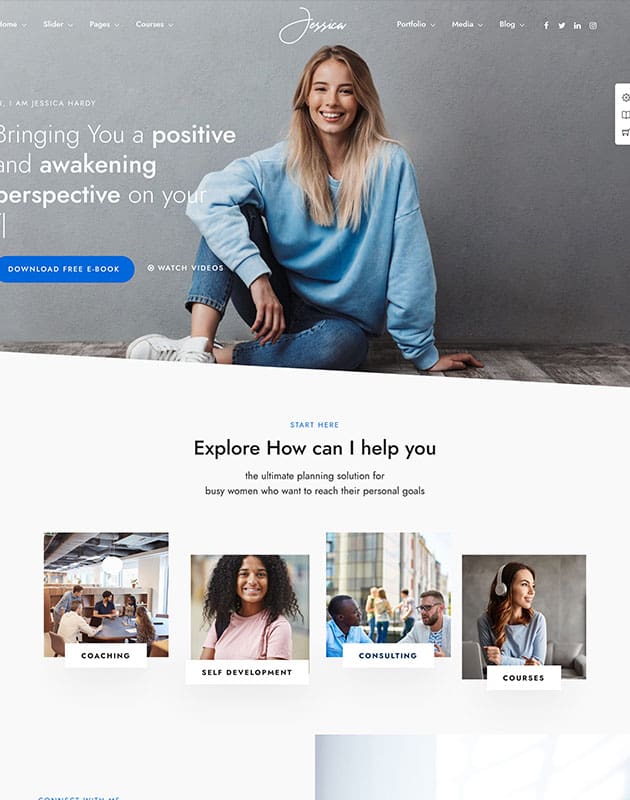The image depicts a promotional section from a website. The background is predominantly grey, with a headshot of a young woman with blonde hair, who is smiling directly at the camera. She is dressed in a blue sweatshirt, blue capri jeans, and white shoes. Above her, in cursive writing, is the name "Jessica."

To the upper left, the navigation bar displays options including "Home," "Slider," "Pages," and "Courses." On the upper right, additional navigation options include "Portfolio," "Media," "Blog," followed by icons representing Facebook, Twitter, LinkedIn, and Instagram.

Below the navigation bar on the right side, there is a white box with grey icons inside showing a gear, a book, and a shopping cart. On the left-hand side, there is a text introduction starting with "I'm Jessica Hardy, bringing you a positive and awakening perspective on your..." but the rest of the text is cut off.

Further down, there is a blue button with white text that reads "Download Free eBook," and adjacent to it, text in black and white indicating "Watch Videos." Below this, on a white background with grey text, the prompt "Start Here" appears, followed by "Explore how I can help you, the ultimate planning solution for busy women who want to reach their personal goals."

The bottom section features four generic stock photos: a meeting scene, a black woman looking straight ahead, a black and white man standing outside deeply engaged in conversation, and a classroom setting where a woman with headphones is looking to the left. In the bottom left corner, there is faint, nearly unreadable text.